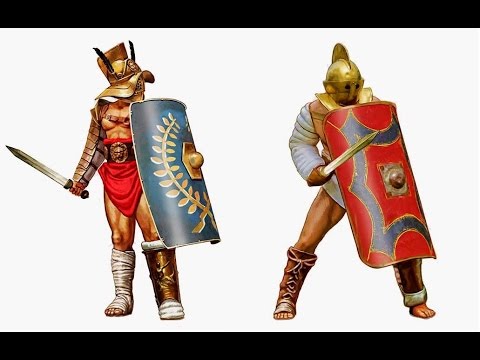This detailed illustration depicts two ornately armored knights standing against a white background with black borders at the top and bottom. The knight on the left, bare-chested except for a necklace, holds a sword in his right hand and a blue shield in his left. His red loincloth is secured with a black belt and a lion-faced buckle. His helmet is distinguished by two black horns and a metal crest with an emblem on the front, an eye shield covers his eyes. His legs contrast sharply; one is wrapped in a white bandage while the other is encased in metal armor. The blue shield features a wreath of leaves flanking a golden knob. The knight, poised to fight, faces the second knight.

The second knight, facing slightly forward, has a golden helmet with a round crest and eye holes. He wears a metal vest over a white tunic and carries a sword in his right hand. His left grips a large red shield, edged with a scalloped blue border and bearing a central knob. Both knights don mismatched footwear; the right knight wears an armored boot on one leg and a lace-up boot on the other, with exposed toes. Their helmets, swords, and contrasting stances – one in an active defensive posture, the other more relaxed – suggest they are either fantastical or historical fighters ready for combat.